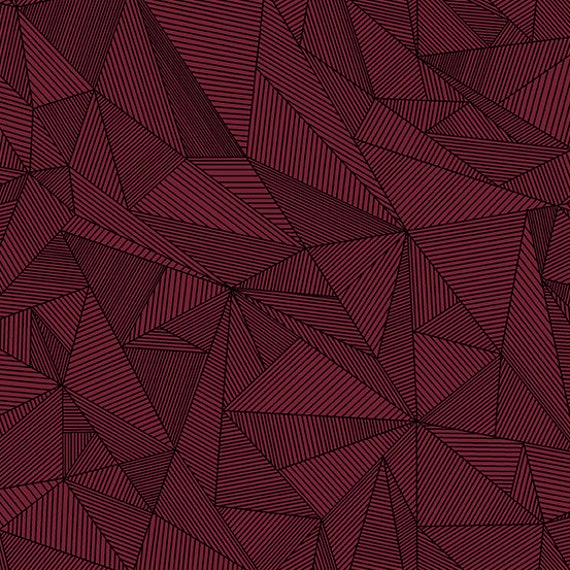The image showcases a complex, digitally generated pattern on a predominantly maroon and black background, characterized by an abundance of triangles in various shapes and sizes. These triangles feature dark lines running either horizontally or vertically, depending on their orientation, creating a sense of chaotic geometry and intricate detail. The red and black interplay, along with the varied angles and the parallel lines within the triangles, conveys a three-dimensional effect, reminiscent of prisms and suggesting dynamic movement. The overall visual impression is one of folded origami-like structures and three-dimensional patterns, making it a uniquely intricate and visually stimulating composition.